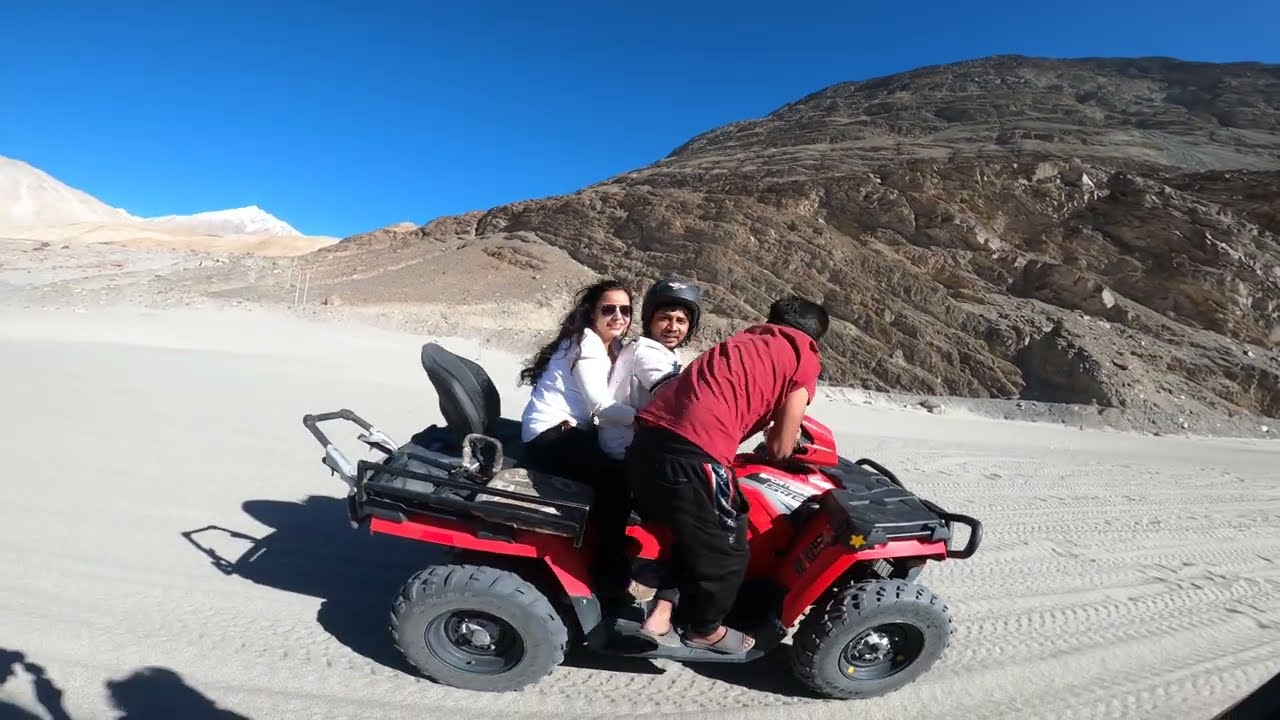The photograph captures a dynamic desert scene featuring three people atop a white and black ATV navigating a sandy road marked with tire tracks, set against the backdrop of a rocky hill or mountain. The clear, cloudless sky transitions from dark to light blue, highlighting the daytime setting. 

The person closest to the front of the ATV is a man wearing a black helmet and a white shirt, driving the vehicle. Behind him is a woman with long black hair, donning black sunglasses, a white long-sleeve shirt, and black pants. Perched on the side footwell of the ATV is another man in a red t-shirt, black sweatpants, and black sandals, leaning over the handlebars.

The detailed terrain features a sandy desert strewn with rocks at the base of the rocky hill. The bottom left of the image shows the shadow of additional people, indicating the presence of others in the vicinity.